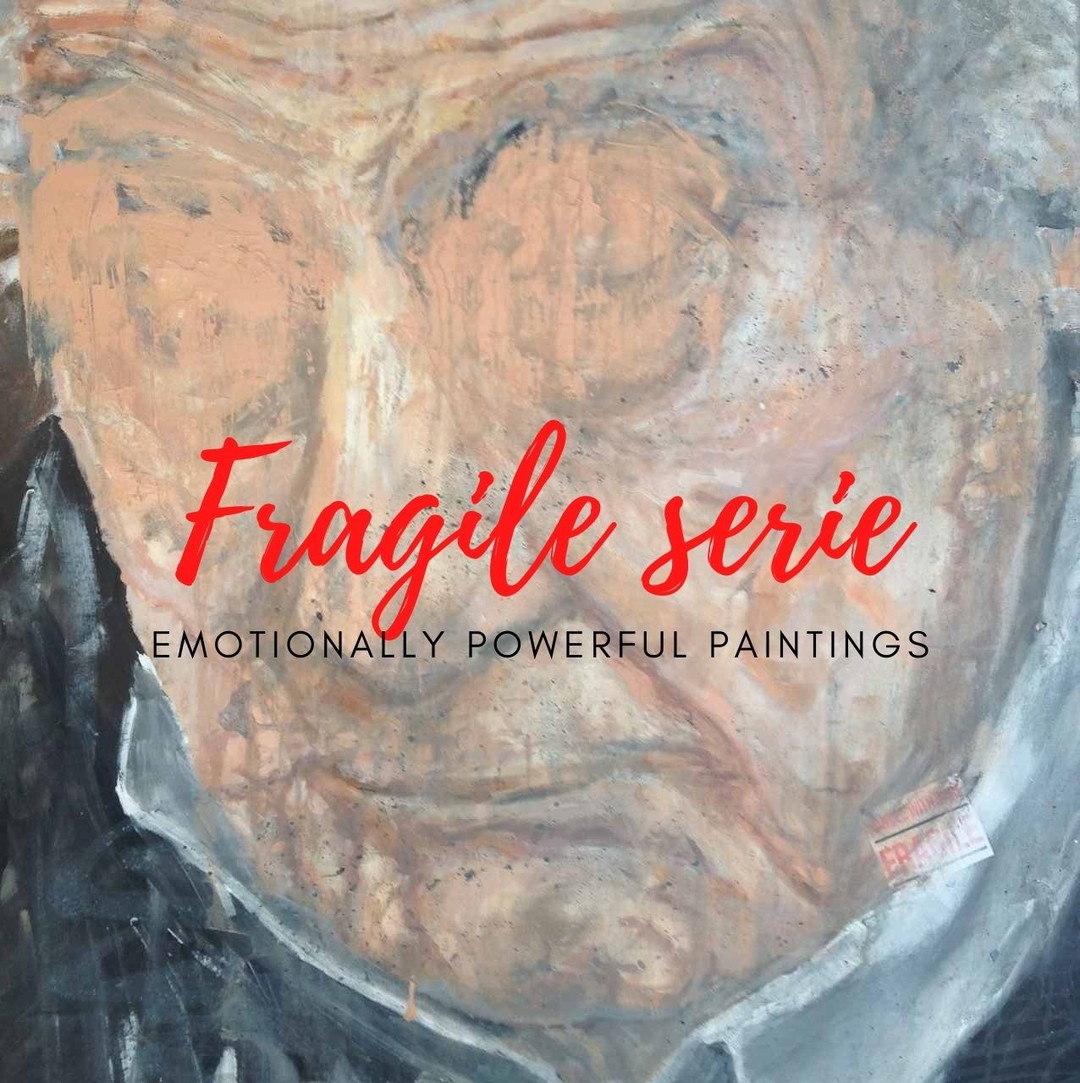The image is a detailed, Impressionist-style close-up of an older man's face, resembling a watercolor painting. His eyes are closed, and you can faintly see his peach-colored skin with noticeable wrinkles on his brow and chin. His eyes appear as large, closed orbs, and his thin nose leads down to fuller lips that remain straight and closed. The man has subtle gray hair in the upper right corner. He is dressed in a white collared shirt with a dark jacket. Prominently featured in the center of the painting is red cursive text reading "Fragile Siri." Beneath this, in smaller, capitalized black text, are the words "Emotionally Powerful Paintings."